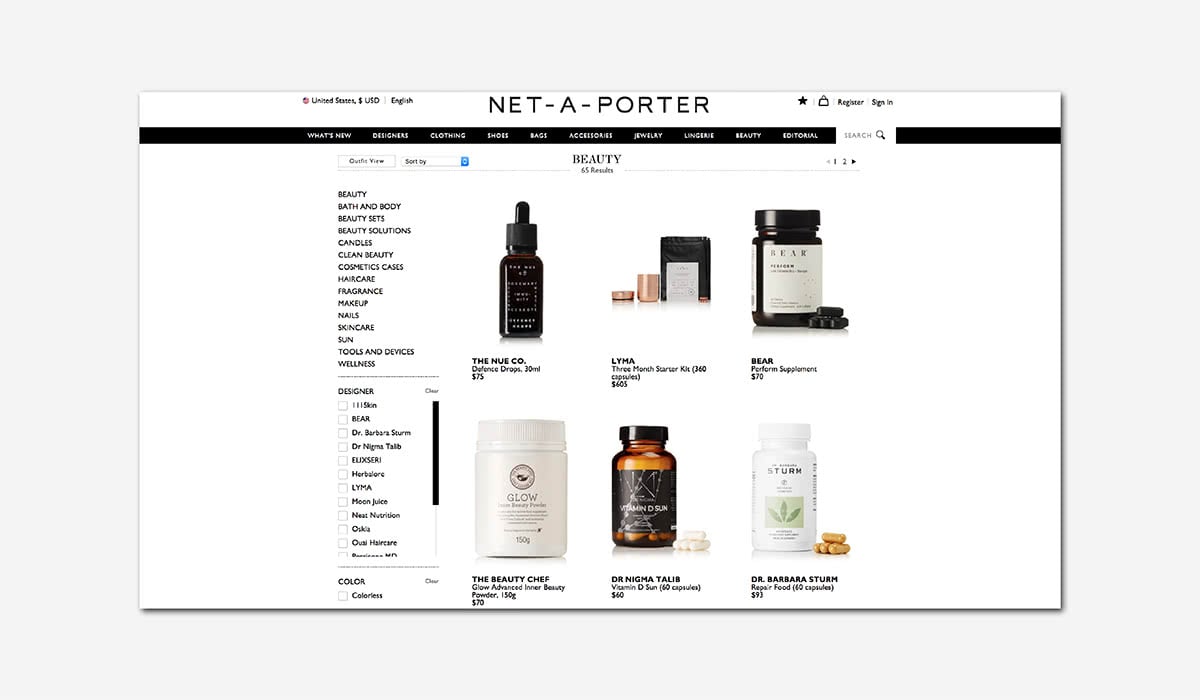A detailed screenshot of a website is displayed with a prominent drop shadow effect, suggesting it may be a mock-up. The top of the page is marked by a black navigation bar containing unreadable menu options. Below this, the word "beauty" is clearly visible. The left side of the screen features a vertical menu listing categories such as beauty sets, candles, cosmetics, cases, fragrance, makeup, nails, and skincare, although the text is somewhat difficult to make out.

The main content area is predominantly white and presents various e-commerce options. On the right side, there are images of skincare products, including an item with a rubber dropper cap likely used for serums, and to its right, makeup products. Further down, there are several bottles and jars containing pills, with labels that are hard to decipher. A black bar featuring an inscription that appears to say "peak" lies just above another section labeled "glow," which contains more pill bottles. The website is identified as Net-A-Porter, with customization options for the United States, US Dollars, and English language settings.